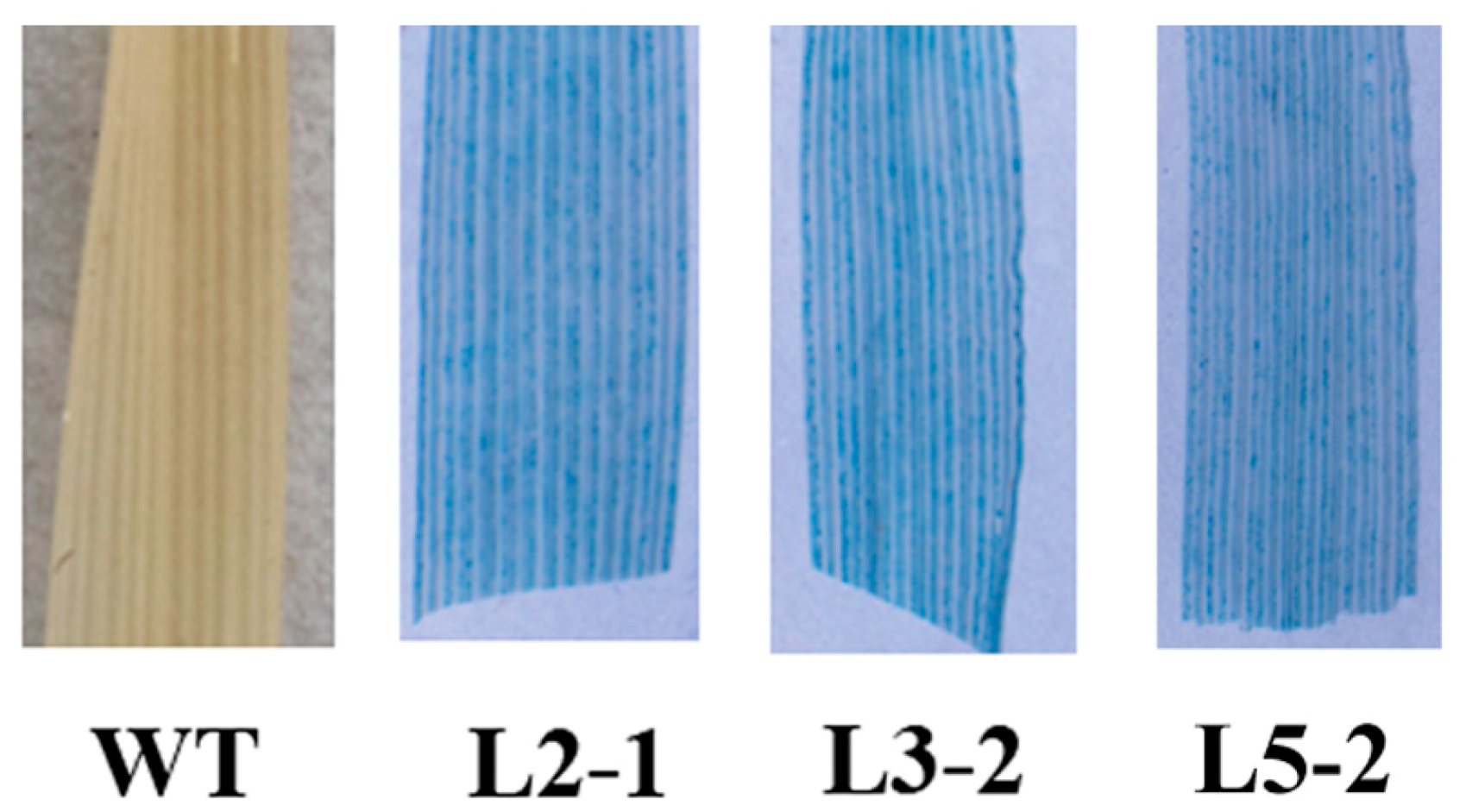This image consists of four vertically aligned rectangular boxes, each displaying a distinct pattern. The boxes are labeled at the bottom: WT, L2-1, L3-2, and L5-2 respectively, from left to right. The far-left rectangle, labeled WT, stands out with an orange and camel color scheme resembling light plywood. The other three rectangles, labeled L2-1, L3-2, and L5-2, share a similar design featuring light blue and white horizontal stripes, and they vary slightly in pattern but maintain the same color palette. The background of the image is gray, creating a neutral backdrop that highlights the differences and similarities among the rectangles.